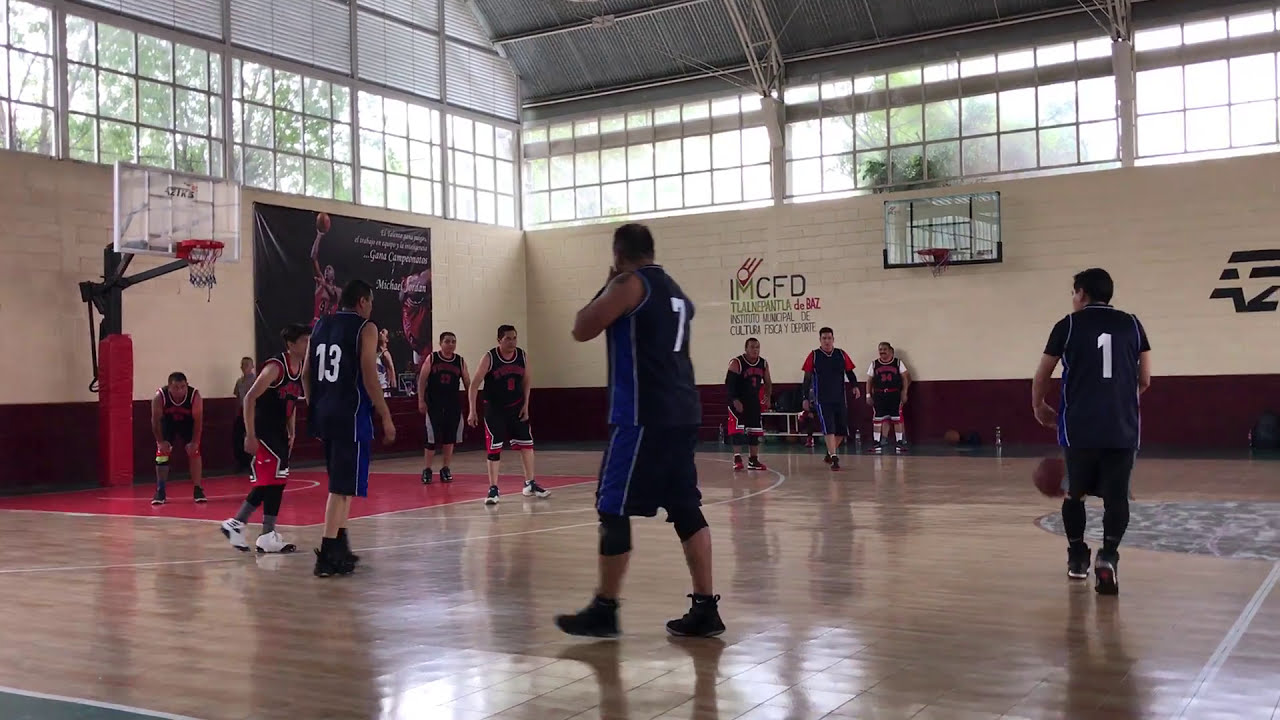This detailed photograph captures an intense moment in a basketball game within an indoor gymnasium. The game features two teams; the defensive team is clad in black and red, while the offensive team sports black with blue accents. The action is centered on a player from the blue team dribbling the ball towards the basket, under which players are strategically positioned. The shiny wooden court glistens under the indoor lighting, reflecting the players' swift movements. Surrounding the court, the gymnasium's white brick walls rise up, adorned with a prominent windowpane that wraps around the top, allowing natural light to filter in and providing a glimpse of the outside trees. Above the playing area, a banner featuring what appears to be Michael Jordan adds a historical touch. On the sides of the court, lettering spells out "IMCFD," potentially signifying the facility or league. Scattered around the court, the vibrant uniforms and the polished tile flooring contribute to the dynamic atmosphere of this mid-day basketball match.